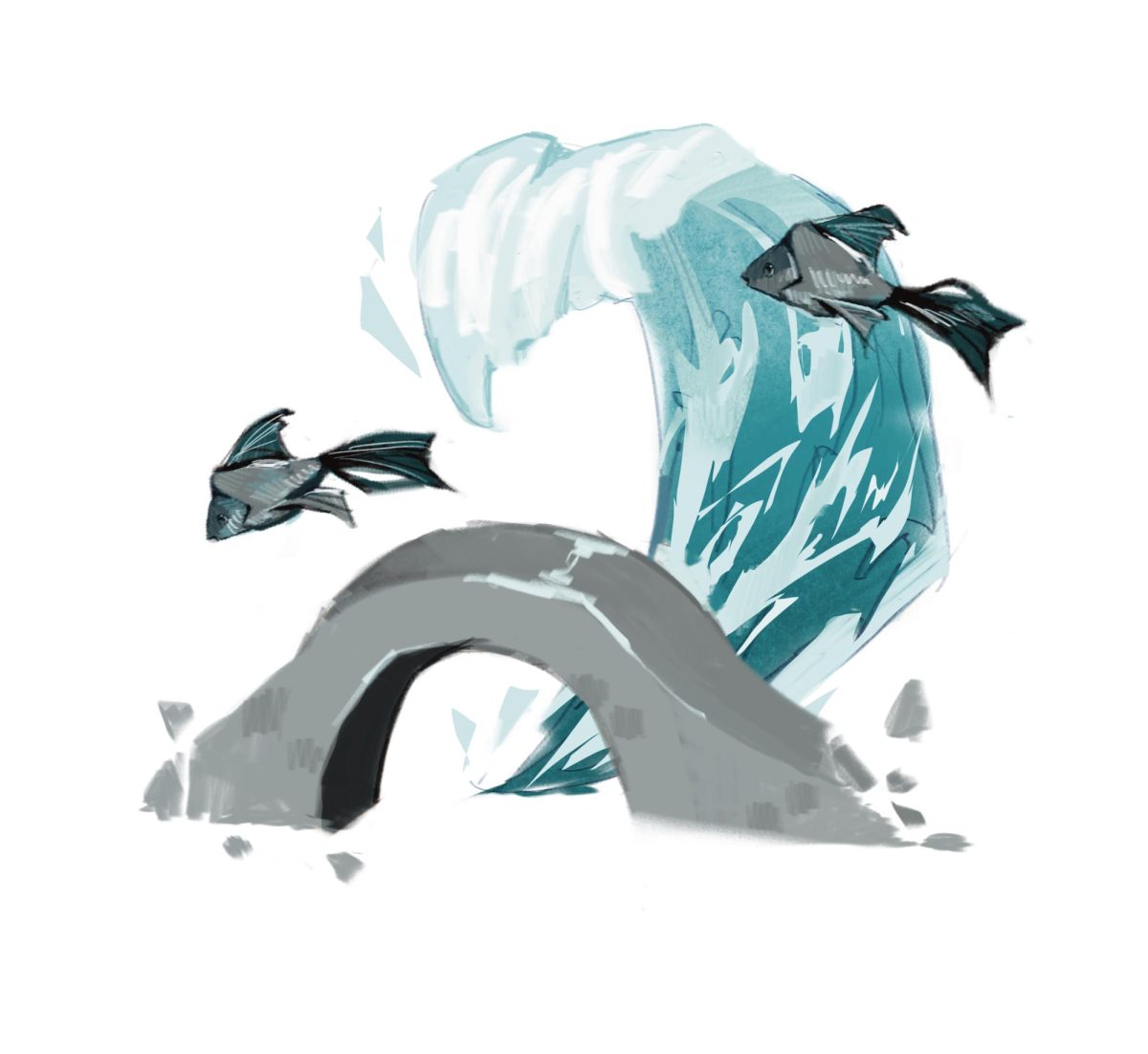This detailed image depicts an abstract digital illustration with a watercolor effect, featuring two large, triangular-shaped fish leaping out of a body of water and soaring through the air. The fish are rendered in shades of dark turquoise blue and gray, with distinct, long tail fins and top fins. One fish has a turquoise blue face with a gray body and side fins, while the other is predominantly gray with turquoise blue tail and top fins.

The scene is set against a simplistic white background, which emphasizes the vivid colors of the fish and water. Beneath the fish is a gray, arch-shaped bridge with a semi-circular opening at its center, reminiscent of a concrete structure. A massive wave, painted in gradients of crystal blue to light blue with white highlights at the crest, looms over the bridge, almost defying the scale of the small stream suggested by the scene. The interplay between the bridge, wave, and fish adds a surreal quality to the artwork, evoking a sense of whimsy and mystery.